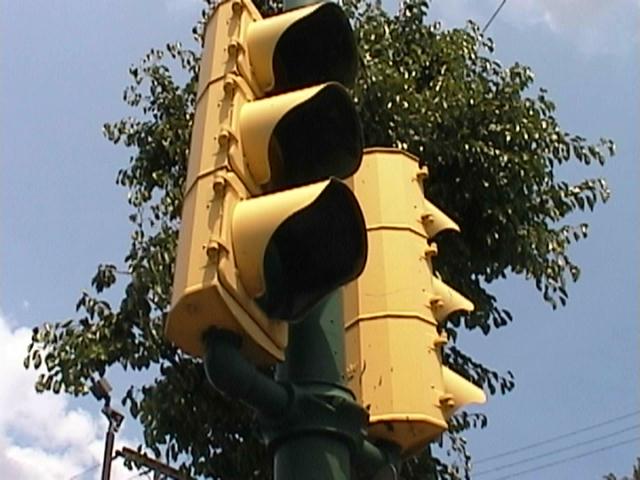In the center of the image, there are two prominent traffic lights mounted on a dark green post. The backdrop features a rounded tree adorned with vibrant green leaves, standing out against a grayish-blue sky. A cluster of clouds occupies the lower left portion of the sky, adding subtle variation to the scene. The traffic lights themselves are encased in a structure painted in a shade of goldish-yellow. The light to the left is oriented toward the right side of the image, with its face slightly angled forward, rendering the lights themselves unseen and casting the enclosure into shadow. The second light, positioned to the right of the first one, points toward the back of the image, directly at the tree, although only the awning portions of its enclosure are visible. On the bottom right corner of the image, three fine lines resembling electrical wires stretch across the scene, contributing to the urban feel of the setting.